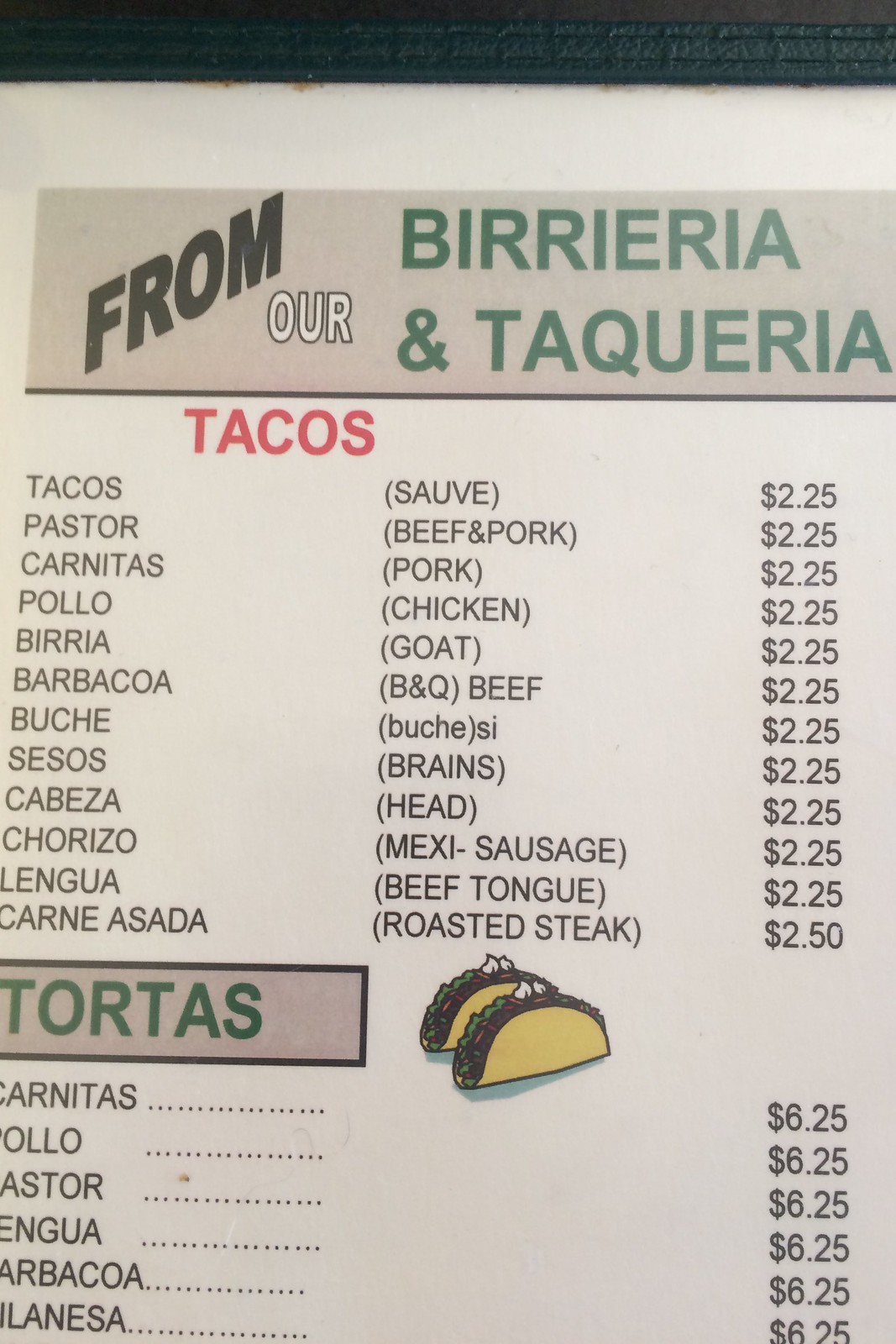The image displays a portion of a restaurant menu, presenting both the name of the establishment and its offerings. At the top, "La Birrera" and "Taquería" are prominently featured, indicating a focus on beverages and taquería-style dishes. Below this heading, the menu items are listed with descriptions in both Spanish and English.

The menu section highlights an assortment of tacos, each with its price indicated. The following taco varieties are displayed, all priced at $2.25 each, unless otherwise noted:

- Tacos Suave (Soft Tacos)
- Pastor (Marinated Pork)
- Beef and Pork
- Pork (Carnitas)
- Chicken (Pollo)
- Goat (Birria)
- Barbecue Beef (Barbacoa)
- Brains (Sesos)
- Head (Cabeza)
- Mexican Sausage (Chorizo)
- Beef Tongue (Lengua)

Additionally, there is an option for "Roasted Steak" (Carne Asada) tacos, which are priced slightly higher at $2.50 each. The text is clearly written in red, making it easy to distinguish the different taco options available.